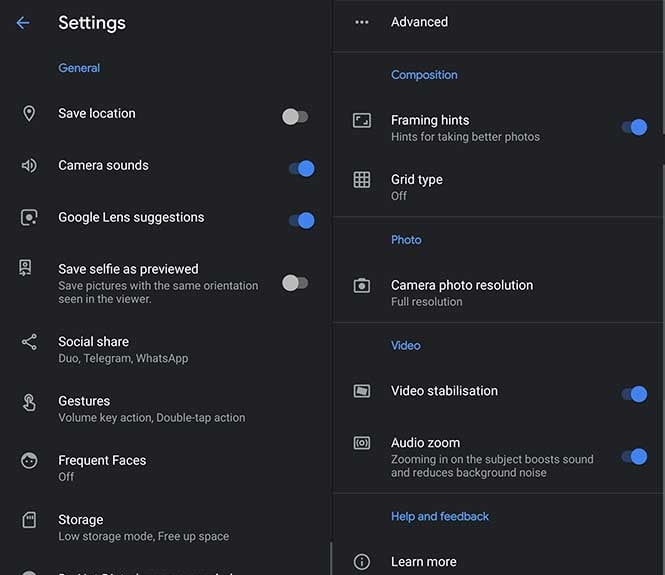The image depicts a dark-themed settings menu from an unidentified device, possibly a mobile or a PC. The settings interface features several options, each accompanied by a toggle switch that turns blue when activated and white when deactivated. Visible settings include "Save Location," "Camera Sounds," "Google Lens Suggestions," "Social Share," "Gestures," "Frequent Faces," and "Storage." To the right, an additional sidebar presents advanced settings for each main option. At the bottom of the menu, a "Learn More" button provides further information about each setting.